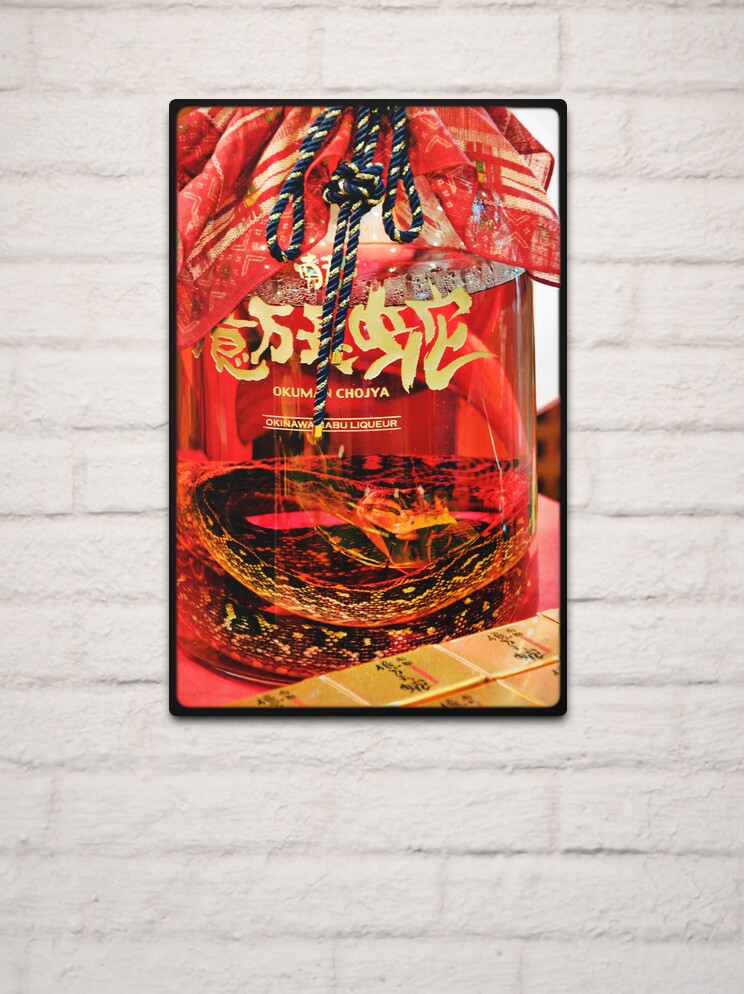The image depicts a framed poster hanging on a white brick wall. The poster itself appears to be an advertisement for snake wine. Central to the photograph is a large, clear bottle featuring a coiled snake at the bottom, poised menacingly. The bottle is adorned with a red and gold cloth at the top, secured by a braided black and gold cord. Prominent gold lettering in what appears to be Japanese or Chinese script decorates the upper part of the bottle. Below this lettering, it reads "Okuman Choja" and "Okinawa Aboa Liquor." Towards the bottom of the photograph, there are gold bars with Asian writing on them, adding an additional layer of detail to this visually rich advertisement.